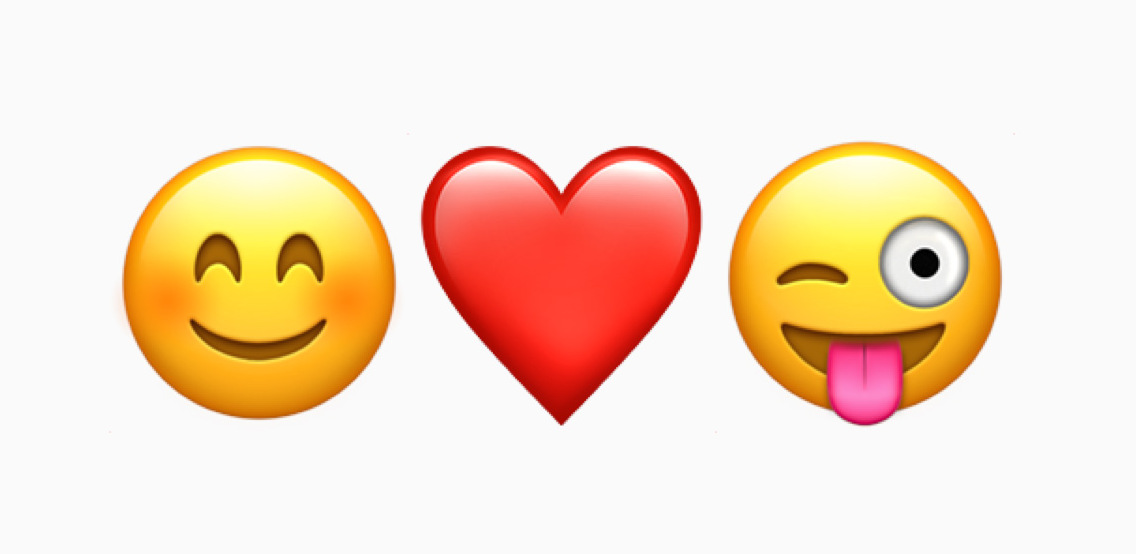On a rectangular, off-white background, there are three familiar emojis arranged horizontally. The leftmost emoji is a round, yellow face with a darkened border and blush-colored cheeks. It has smiling, crescent-shaped eyes that curve downward and a thin, crescent-shaped smile curving upwards. In the center is a large, red heart with white highlights at the top, as if reflecting sunlight. The rightmost emoji is a playful, yellow face with an orange-shaded perimeter. It has one large, wide-open white eye with a black pupil and the other eye is a closed crescent, giving a winking effect. Its mouth is open, showcasing a tongue that is pink in the center and purple towards the edges.